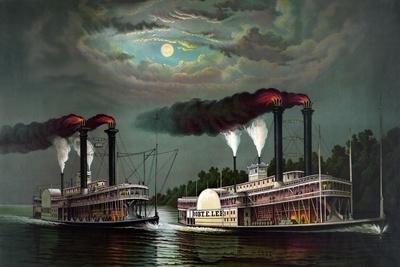This detailed illustration depicts a twilight maritime scene featuring two steamboats navigating a shadowy, swamp-like river. The painting captures the larger steamboat slightly ahead and to the right, while a smaller one trails behind to the left. Both vessels are primarily white with hints of pink and are characterized by their tall stacks—each boat having two stacks emitting voluminous smoke. The billows transition from yellow near the pipes to red, then black, and finally fade to blue as they ascend, creating a dramatic visual effect. Surrounding the boats, dark, swirling clouds dominate the sky, coalescing into a near-perfect circle with a striking white full moon or almost-full moon at its center, visible through the eye-like gap in the otherwise tumultuous storm clouds. This central moon and the stormy clouds contribute an eerie ambiance to the scene. Adjacent to the riverbank, a dense line of trees further enhances the image's haunting allure. Overall, the contrast of the illuminated moon, shadowy smoke, and serene yet ominous water creates an evocative and atmospheric portrayal of these two steamboats caught under a tumultuous sky.